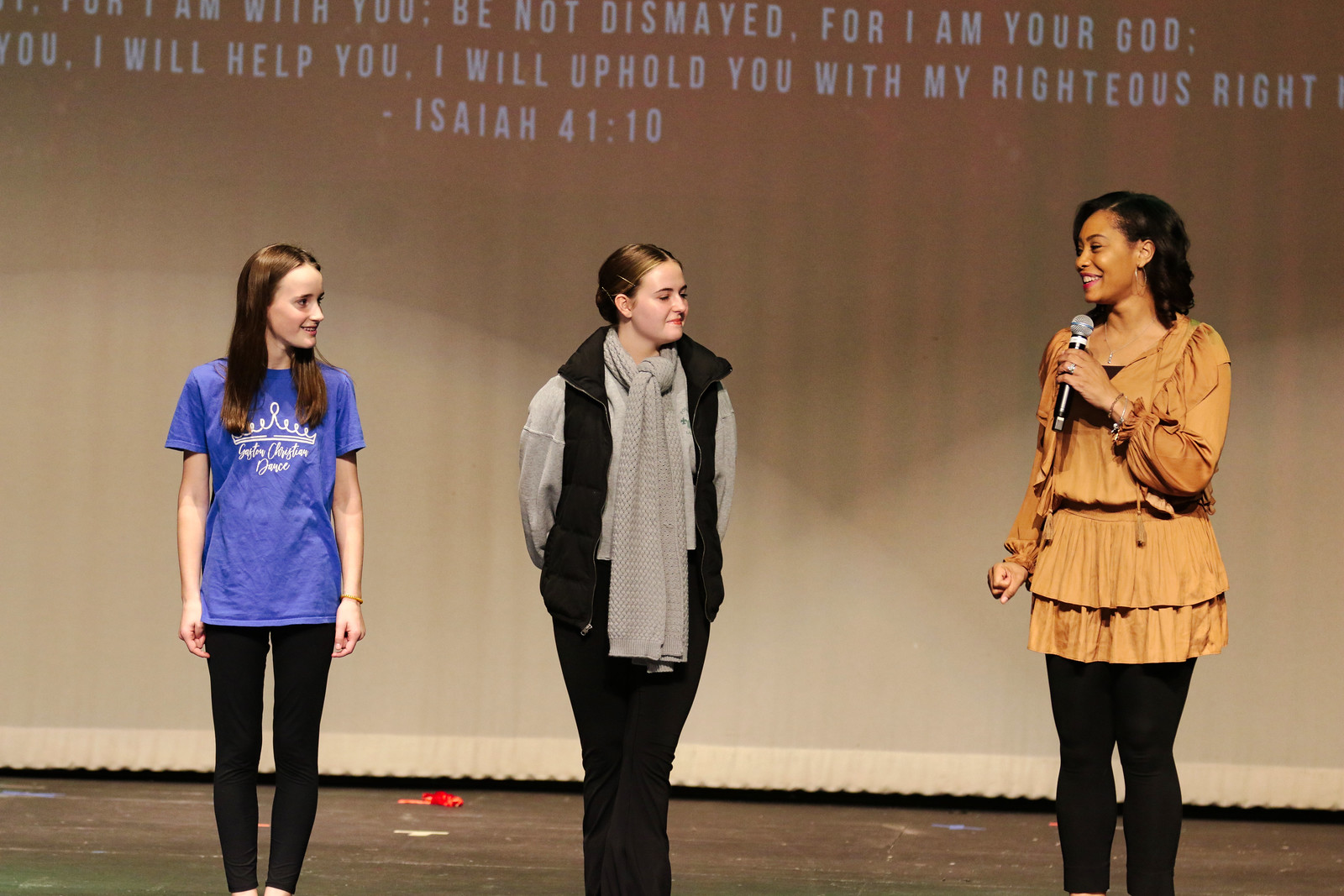This image captures a scene on stage with three women under a backdrop displaying a partially visible Bible verse from Isaiah 41:10. The woman on the right, who appears to be the host, is a black woman with shoulder-length curly hair. She is smiling and holding a microphone in her left hand, wearing a dark tan or brown top paired with black pants. To her left, a white woman stands with her hands behind her back, smiling with her eyes closed, and has smooth brown hair. She is dressed in a black vest over a black top, accessorized with a gray scarf, and wears black pants. The other white woman, positioned on the far left, has chest-length brown hair and open eyes. She is clad in a blue t-shirt with an indiscernible logo and black pants. The stage curtain behind them bears the biblical text, “Isaiah 41:10: Do not fear, for I am with you; do not be dismayed, for I am your God. I will strengthen you and help you; I will uphold you with my righteous right hand,” though the top part of the quote is slightly cut off.